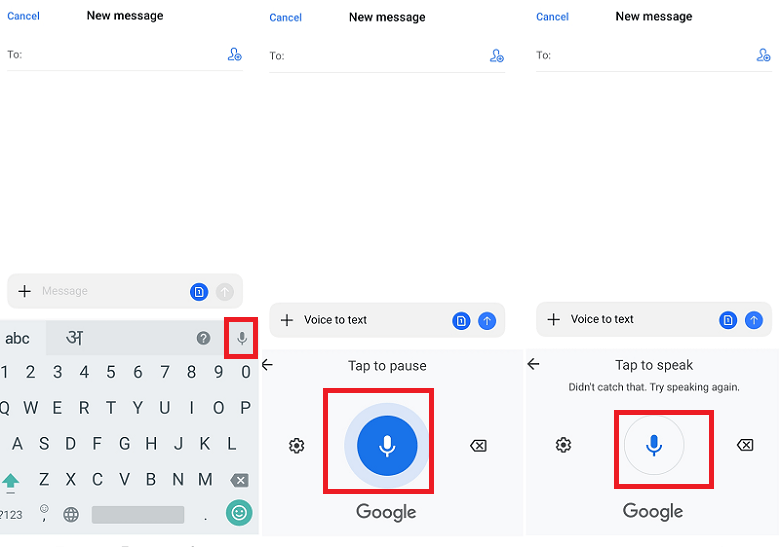**Caption:**

Under the heading "Webpages," the image sequence displays three new message screens, all in the initial stages of composing a message.

1. **First Screen**: Each screen is blank with the header, "New Message" in black letters and a "Cancel" option in blue. The recipient field remains empty, symbolized by an icon of a person’s head and shoulders. At the bottom, there's a plus sign labeled "Message," above a visible keyboard with basic letters and a settings button.

2. **Second Screen**: Identical to the first screen in layout, but enhanced with a voice-to-text feature at the bottom. A blue circle containing a white microphone icon is enclosed in a red box labeled "Tap to pause," indicating active voice recording.

3. **Third Screen**: Similar to the first screen, but under the voice-to-text feature a message reads, "Didn't catch that, try speaking again," indicating an issue with the voice input.

This series comprehensively illustrates the interfaces and options within the new message composition feature on a webpage.